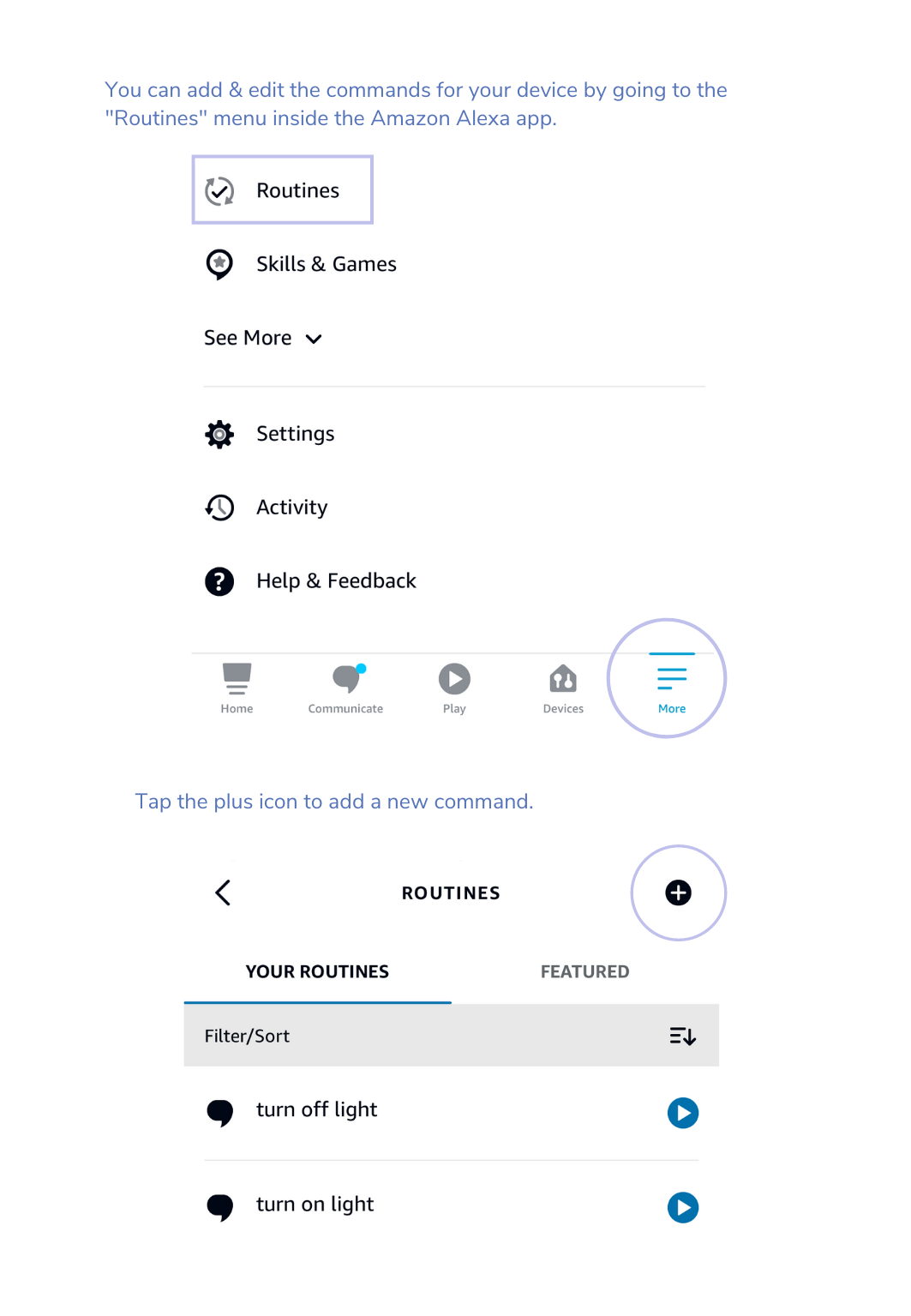The screenshot depicts the "Routines" menu within the Amazon Alexa app, highlighting the functionality for adding and editing device commands. At the top, a message informs users that they can manage their commands by navigating to the routines menu within the app. The "Routines" tab is visually emphasized with a blue box, suggesting either a current selection or an instructional highlight.

Directly below the "Routines" tab are additional sections including "Skills & Games" and a "See More" dropdown menu. Upon expanding this dropdown, options for "Settings," "Activity," and "Help & Feedback" become visible. A thin divider separates these options from the main navigation icons along the bottom of the screen: "Home," "Communicate," "Play," "Devices," and a "More" menu, which is also encircled in blue, possibly as part of the instructional guide.

Within the "Routines" section, users are prompted to tap a plus icon, located at the top, to add a new command. This plus icon, reminiscent of adding a contact on a phone, is also highlighted in blue. The interface showcases an active selection of "Your Routines" over "Featured," with options to filter and sort the routines. Examples of available routines include turning lights on or off.